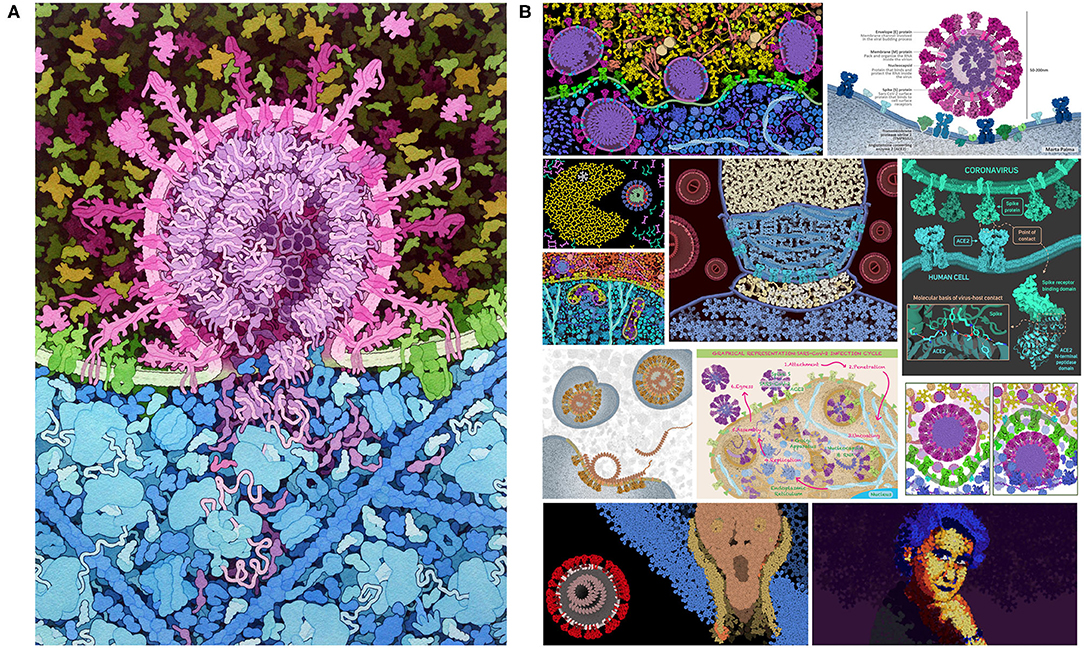The artwork appears to be a poster divided into two sections, labeled A and B. Section A features a predominantly pink circular centerpiece with ornate stem-like extensions. Surrounding these stems is a dark green background adorned with falling leaves in tan, olive green, and lighter green hues. At the base, the poster transitions into a darker blue background interspersed with light blue orbs, which resemble abstract flowers, connected by pink squiggly lines.

Section B consists of multiple smaller panels arranged in a structured layout. The top row contains two panels, followed by a larger central panel flanked by two smaller panels on the right. The next row has three images across, with the central one appearing to be a chart with minuscule text. The bottom row features an image on the left of a man with his hands on his face, reminiscent of the painting "The Scream," set against a dark background with a blue sash-like element. On the right, a woman looks directly at the viewer, resting her chin on her hand, set against a deep violet or magenta background with blue hair. The entire section B is rendered in a pixelated and colorful illustration style, with a blend of abstract and recognizable imagery, including a Pac-Man reference and other intricate designs.